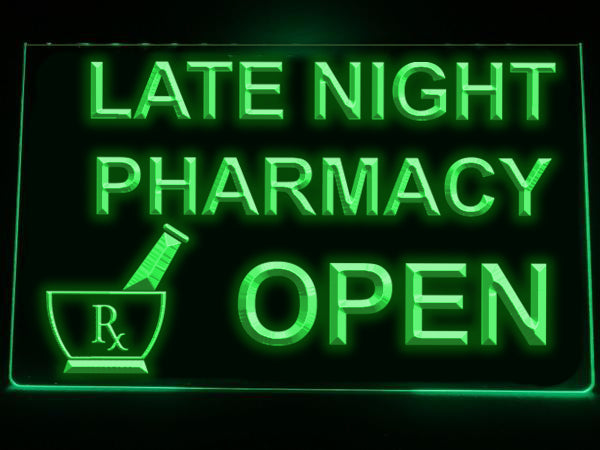The image showcases a vibrant neon business sign against a solid black background, creating a stark contrast that emphasizes its bright, luminous features. The sign is rendered entirely in neon green and forms a square shape. The text on the sign is in bold, uppercase letters and is arranged in three rows. The top row reads "LATE NIGHT," the middle row displays "PHARMACY," and the bottom row, in slightly larger font, states "OPEN." In the bottom left corner, there is a detailed neon depiction of a mortar and pestle, a traditional tool used for grinding pills. The pestle emerges from the bowl, and the bowl prominently features the "RX" symbol, where the 'R' extends into the 'X.' The image's neon elements vary in hue from darker green on the left to a lighter green on the right, possibly suggesting a reflection from a light source. This sign, likely affixed to a pharmacy window, glows vividly amidst the night, indicating that the pharmacy is open during late hours.